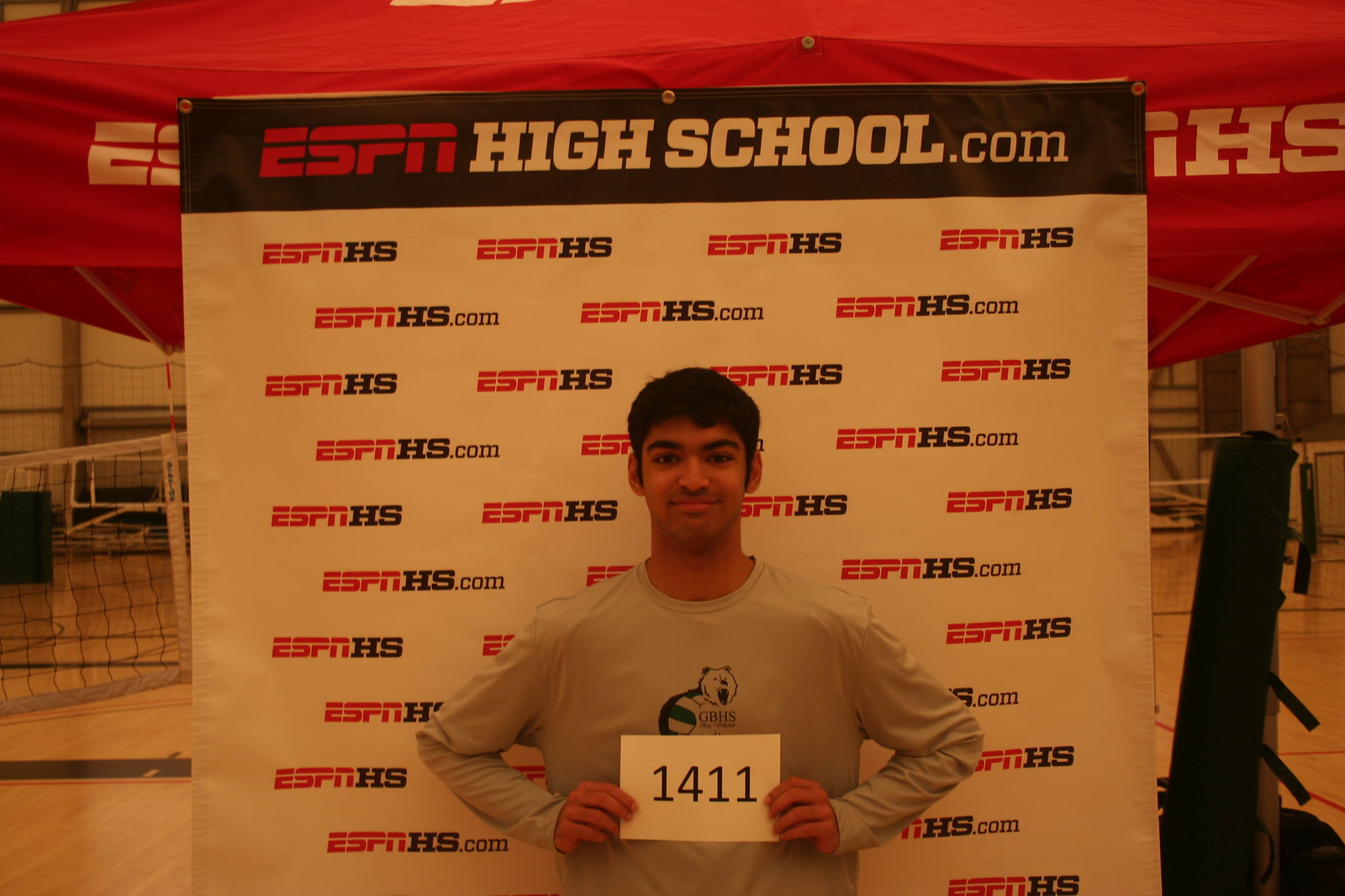In this image taken inside a gymnasium, a teenage boy with a dark complexion and short dark hair is standing in front of a promotional backdrop designed for a sporting event. He's wearing a long-sleeved gray shirt that features the letters GBHS along with a mascot logo, which appears to be a bug with a bear face. The backdrop behind him prominently displays the logo ESPNHIGHSCHOOL.COM and the repeated text ESPNHHS.COM in red and black. The boy is smiling and holding a white piece of paper with the numbers 1411 written on it. The gymnasium setting is evident with visible court flooring and a net in the background, possibly indicating a sport like volleyball.